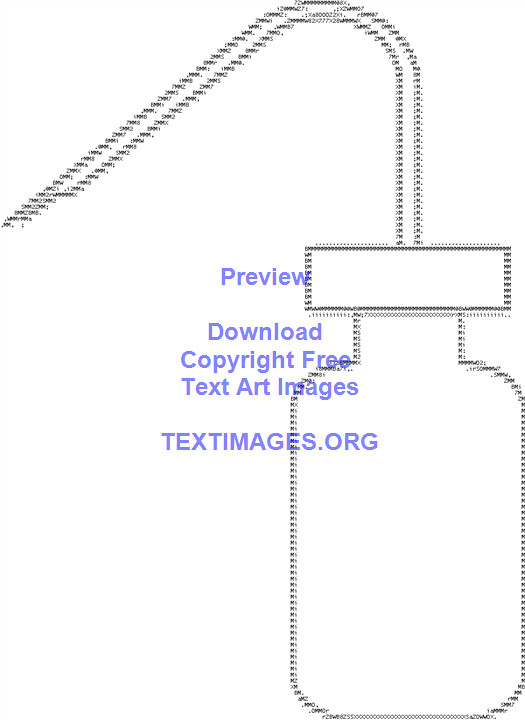The image depicts a clipart of a white bottle with a rectangular top and a spout, resembling a medical or squeeze bottle. It has a distinct black outline and is created using a series of small letters, numbers, or possibly dotted lines. A small hose emerges from the top of the bottle, curving up and to the left before descending again. To the left of the bottle, the word "PREVIEW" is visible in blue letters. Along the neck of the bottle, "DOWNLOAD" is written, followed by "COPYRIGHT FREE" beneath it, with the word "FREE" partially superimposed onto the bottle. Further down, the phrase "TEXT ART IMAGES" appears, with the word "IMAGES" slightly intruding into the bottle's outline. At the bottom, separated by a space, the website "TEXTIMAGES.ORG" is indicated, with portions of the text extending inside the bottle. All these textual elements are rendered in blue.